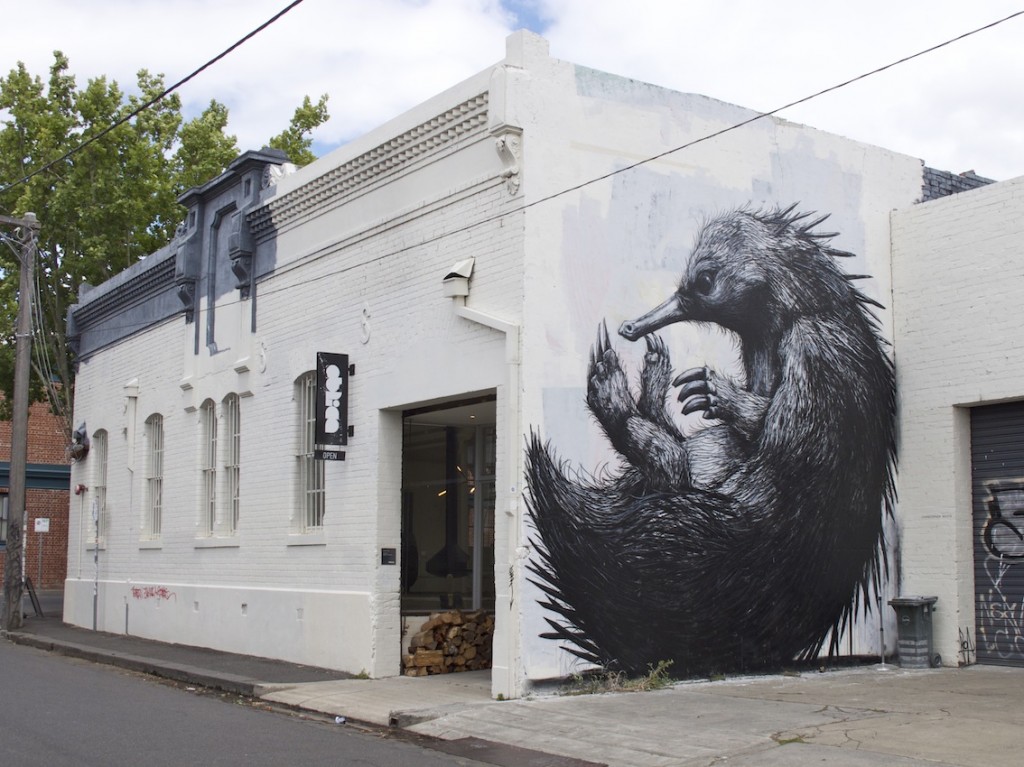This photograph showcases an urban building painted predominantly in white, with its upper left corner featuring a section painted gray. The structure appears to be a shop or restaurant, indicated by an "open" sign on a blackboard positioned near an open door. The front facade is adorned with intricately designed windows, and inside, large glass windows and visible wooden logs can be seen, suggesting ongoing construction.

The building's right side wall is dominated by a striking black and white mural of a large, detailed porcupine. The animal is depicted sitting, with its sharp claws and long, pointy beak prominently visible amidst its shaggy fur. Adjacent to this wall is a closed shutter door, also featuring some unclear graffiti.

In front of the building lies a pavement bordering a green-colored road, with an electric pole and wires prominently standing. Beyond the structure, there is a glimpse of trees and neighboring brick buildings. The sky above is brightly blue, scattered with numerous white clouds, completing the photograph's vibrant daylight setting.